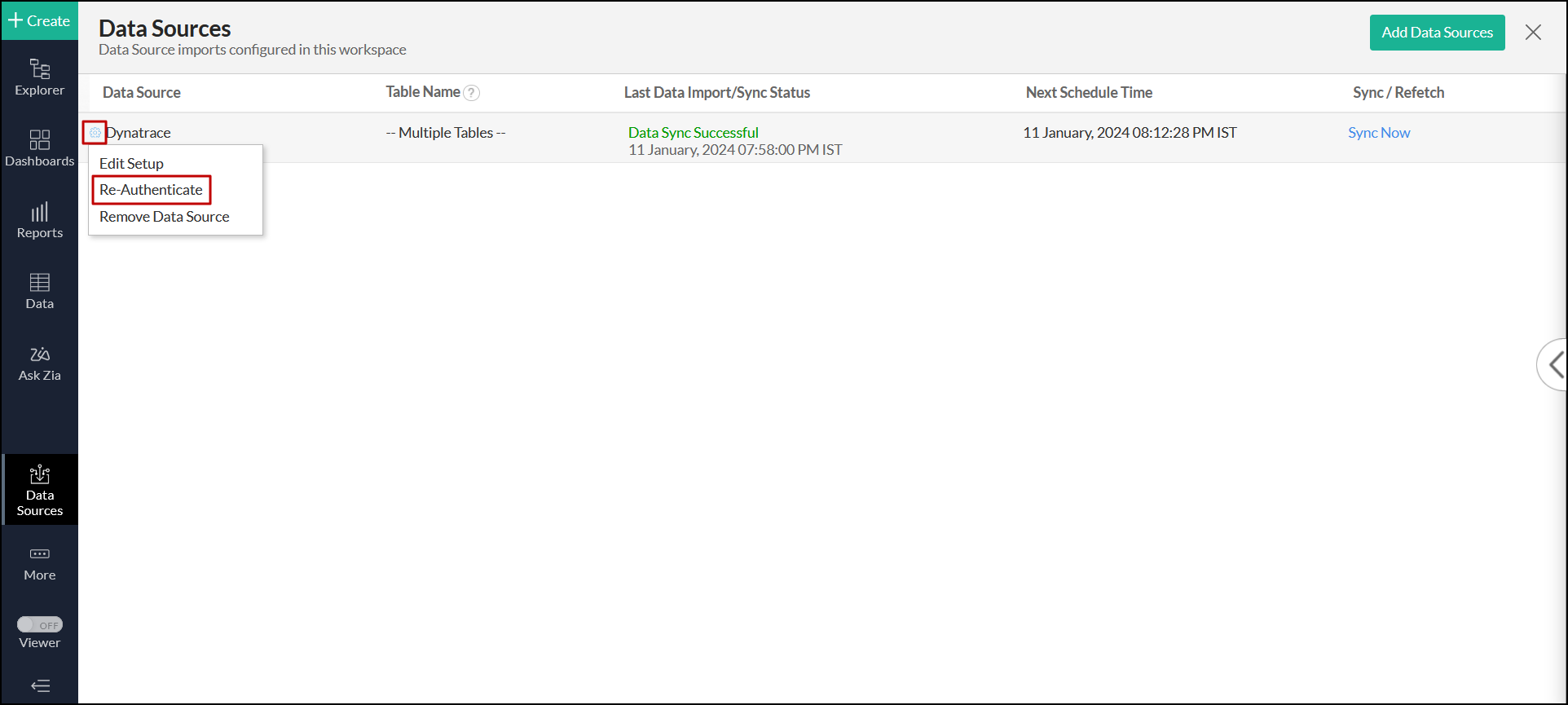The image is a screenshot of a data import platform interface. It is rectangular with a thin black border running along its perimeter. On the left side, there is a vertical dark gray sidebar. At the top of this sidebar, there is a green "Create" button with a plus sign on it. Below the "Create" button, there are several navigation options including "Explore," "Dashboards," "Reports," "Data," and "Ask Zia," which features the word "Zia" in a sleek, single-line font. Below these options is a small black box labeled "Data Sources," under which appears a "More" option alongside a gray toggled-off viewer button.

The top of the main interface features a horizontal gray bar with the title "Data Sources" in black text on the left side. This bar indicates that "Data source imports configured in this workspace." On the right side of this bar is a green "Add Data Sources" button. Directly below this bar is a table header that reads "Data Source, Table Name, Last Data Import/Sync Status, Next Schedule Time, Sync Refresh."

One data source entry within the table is highlighted in red. This entry includes a drop-down menu with options to "Edit Setup," "Re-authenticate," and "Remove Data Source," the latter of which is highlighted in a red rectangle.